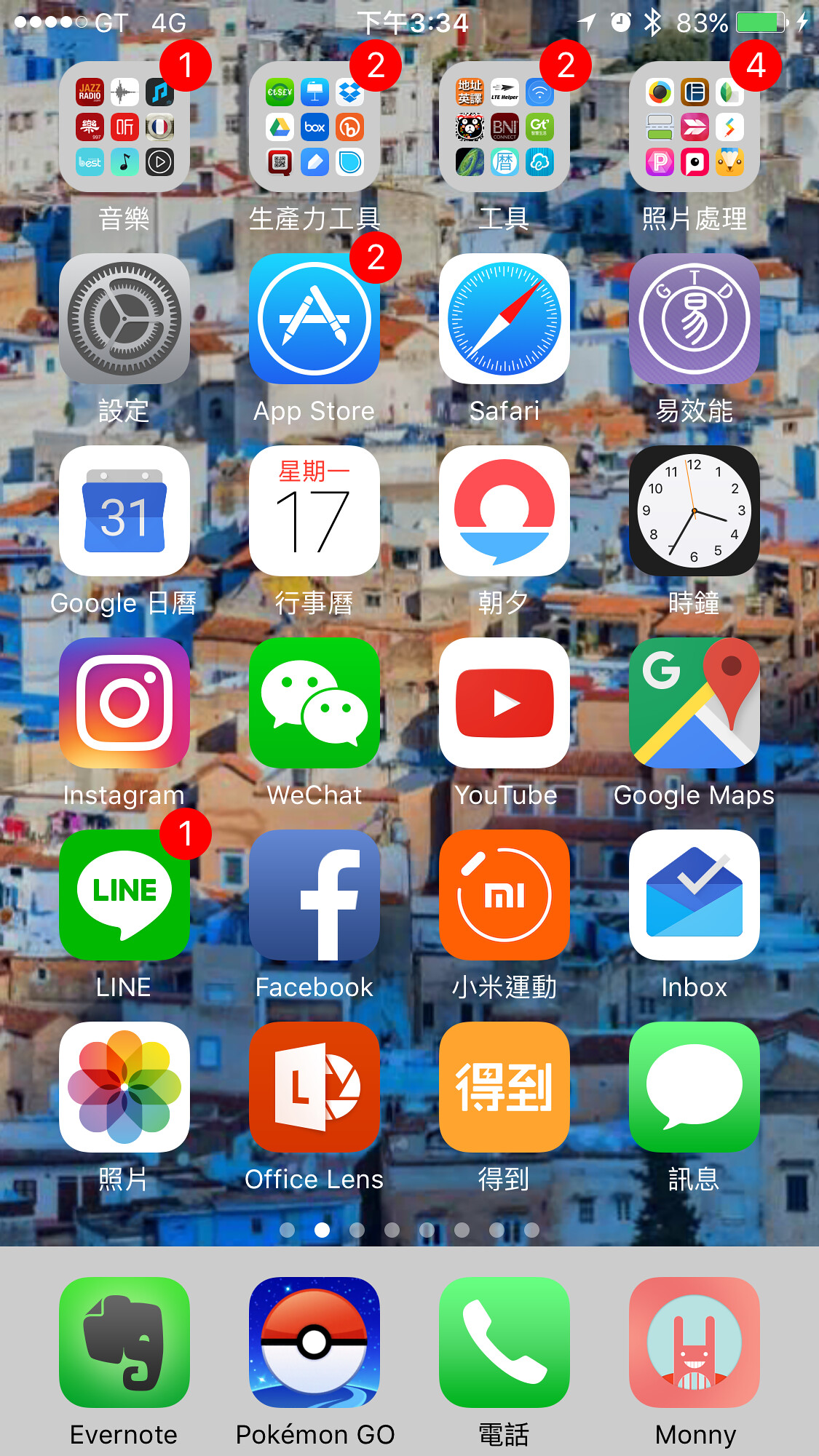This image is a screenshot of a mobile phone's home screen, densely packed with various app icons. The user appears to be Chinese, as many of the apps feature Chinese characters beneath their icons. The phone's background displays a stunning sunset scene, overlooking a densely packed village filled with numerous small houses.

At the top of the screenshot, the status bar is visible. Starting from the left, it shows a 4G connectivity icon, a series of four white dots, indicating an active network, followed by the time in the center. Moving to the right, there's a location symbol, a clock symbol, a Bluetooth icon, a battery percentage of 83% in white text, and finally, a fully charged battery icon in green.

The home screen is organized into four columns and six rows of apps, making for a total of 24 visible icons. The top four icons are folders containing even more apps. Notable app icons on the screen include YouTube, Instagram, Safari, Facebook, and Office Lens, among others. 

Overall, the image captures a detailed glimpse into the user's phone setup, highlighting both the functional and aesthetic elements of their device.